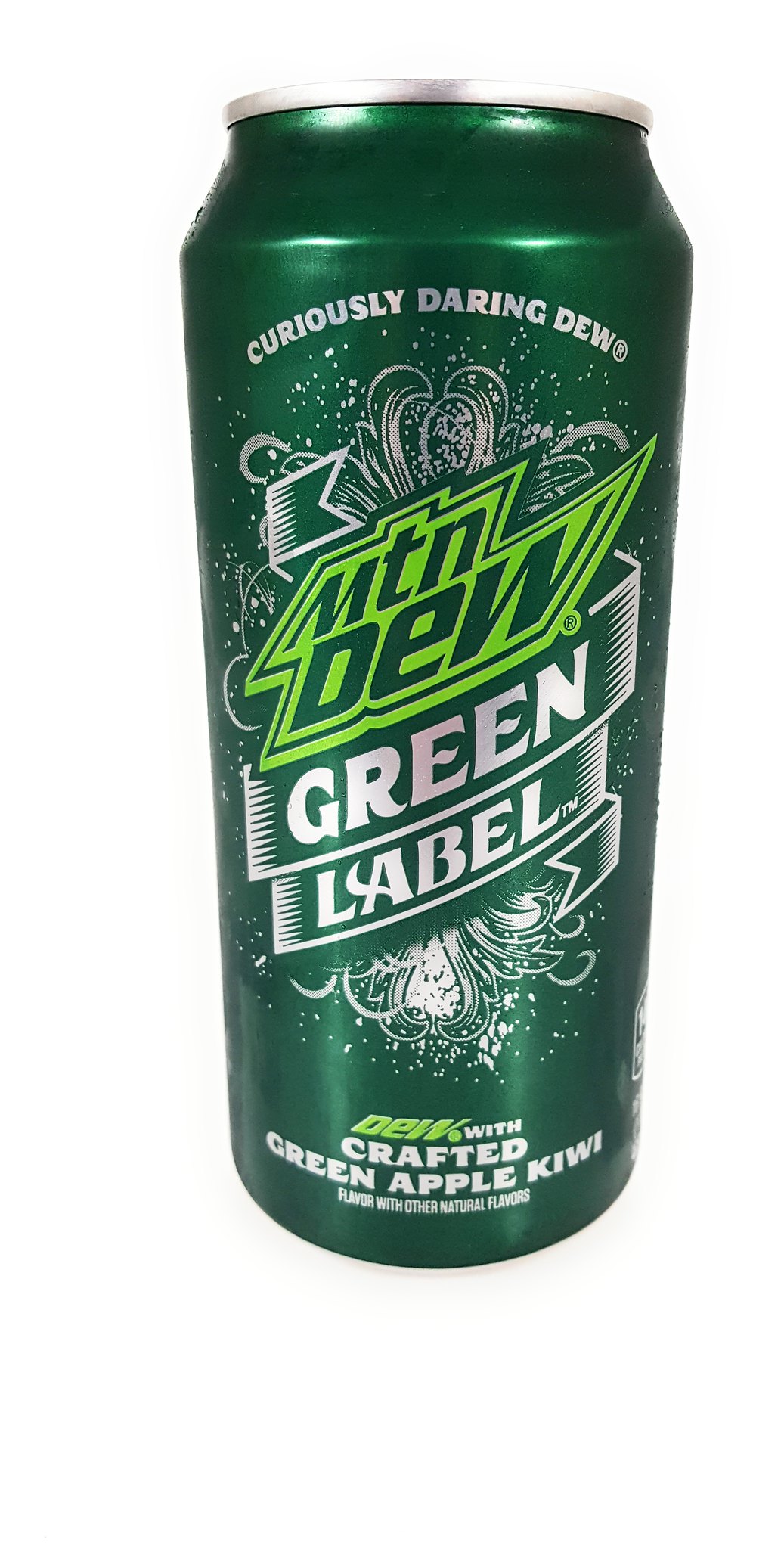This image showcases a sleek, tall soda can set against a plain white background. The can prominently features the "Mountain Dew Green Label" branding at the top and is adorned with the slogan "Curiously Daring Dew" at the bottom. This particular variety boasts a carefully crafted green apple kiwi flavor, complemented by other natural flavors. The can itself is a dark green color, with a silver top and striking silver text. The central label of "Mountain Dew" is highlighted with bright green accents. The background of the design is intricate, featuring subtle patterns that resemble small flowers and dots, adding a layer of sophistication to the overall look. The can's height and shape are reminiscent of typical energy drink cans, adding to its bold and adventurous aesthetic.